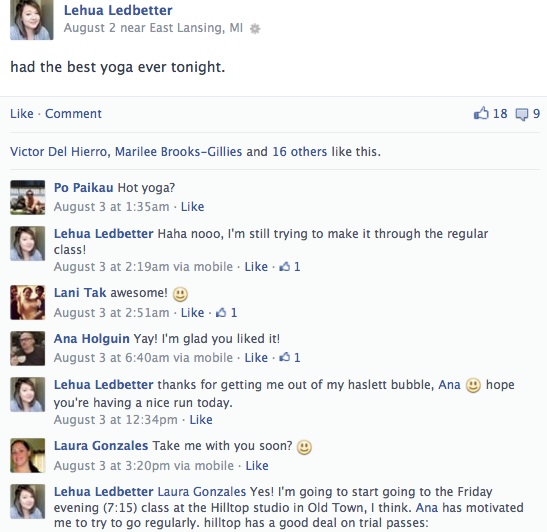The image depicts a Facebook interaction involving Lihar Ledbetter, who posted a status update on August 2nd near East Lansing, MI. The top left of the post shows a photograph of Lihar, a woman with brown hair reaching her upper chest, wearing a blue top. Her status reads, "Had the best yoga ever tonight." This post has garnered 18 thumbs-up and 9 message replies, with Victor Del Hero, Marielle Brooks Gillies, and 16 others liking it.

Below the status, a thread of comments follows:
- Paul Peichold asks, "Hot yoga?"
- Lihar humorously replies, "Haha, no, I'm still trying to make it through the regular class."
- Another user comments, "Awesome, glad you liked it," with Lihar thanking Anna for getting her out of her Hazlit bubble and hoping Anna had enjoyed her run.
- Another comment, "Take me with you soon," invites Lihar's response: "Laura Gonzalez, yes, I'm going to start going to the Friday evening, 7:15 class at the Hilltop Studio in Old Town. Anna has motivated me to try to go regularly; Hilltop has a good deal on trial passes."

This detailed caption captures the essence of the friendly and motivational conversation surrounding Lihar's engaging post about her positive yoga experience.